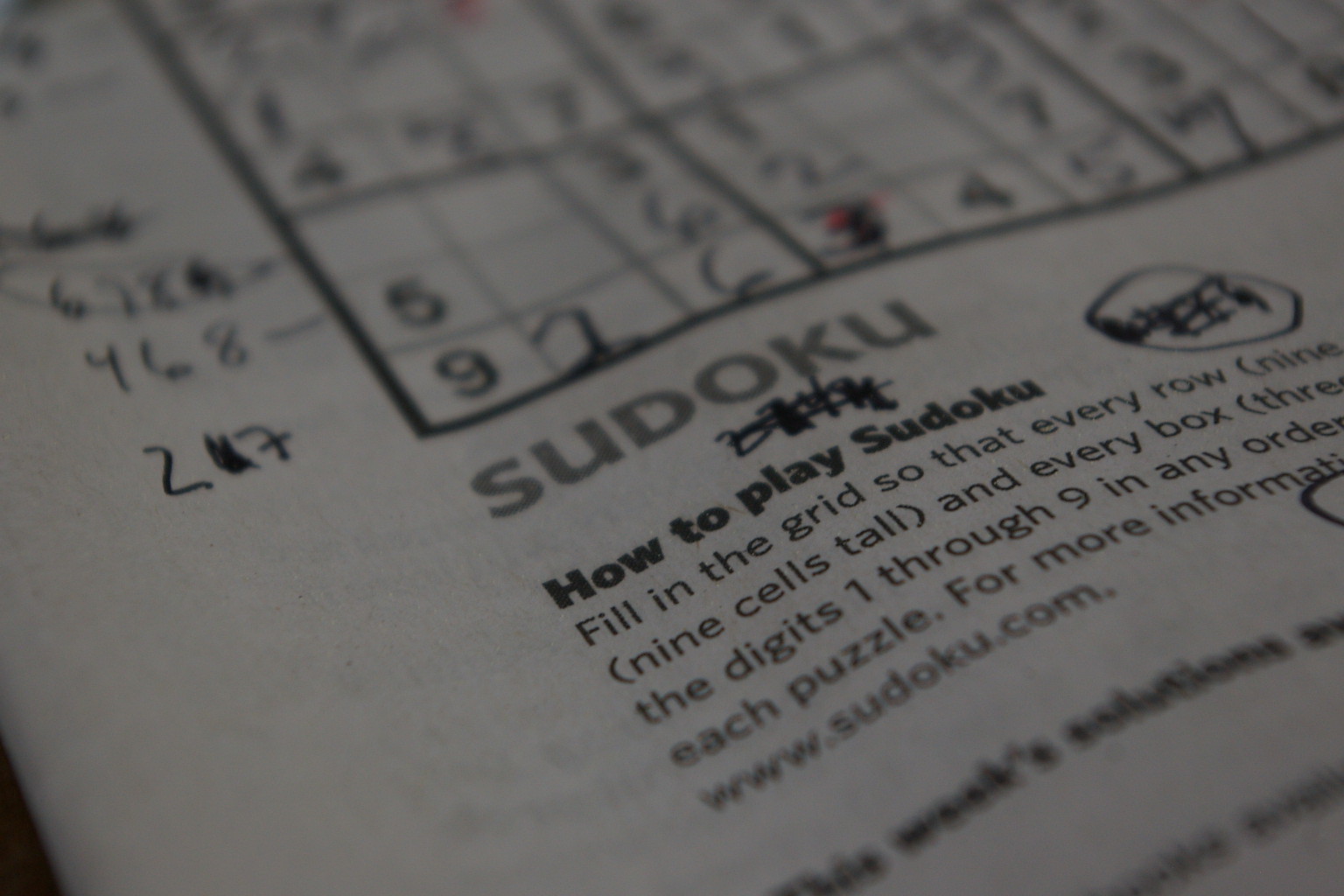This image is a close-up of a partially filled Sudoku puzzle, showing the lower portion of the board. The bottom row is completely filled in with the numbers 9, 1, 6, 3, 4, 5, and 7, with some numbers pre-printed and others handwritten by the solver. The grid features black and grey text, including a title "Sudoku" in grey, followed by a bold black instruction header "How to play Sudoku." Detailed instructions underneath explain how each row (9 cells tall) and each 3x3 box should contain the digits 1 through 9 in any order. Additional text directs to "www.sudoku.com" for more information, though parts of the text are cut off or blurred. On the left side of the image, outside the Sudoku grid, several numbers (2 and 7) are noted on a piece of paper, likely used by the solver for reference or exclusion. The image mainly focuses on the lower segment of the Sudoku puzzle, in black and white.